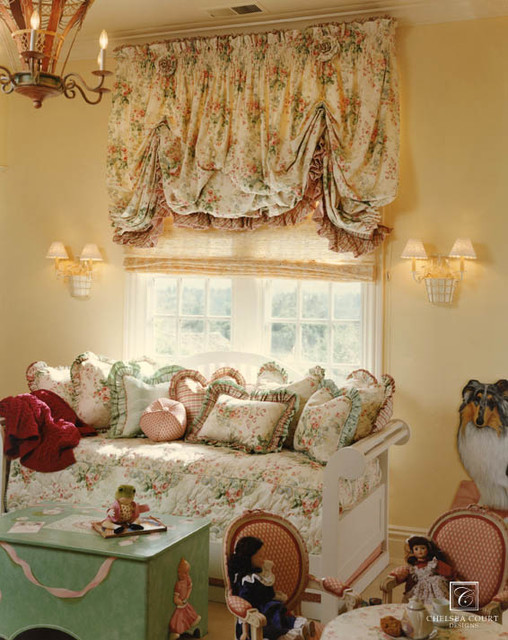The photograph captures a cozy, light-filled child's bedroom, designed for comfort and play. Centered in the room is a large, white loveseat or wooden bench, overflowing with an array of fluffy, frilled pillows in cream, various shades of green, light pink, and adorned with floral patterns, all directly in front of a large double-pane window. The window, with its cream-colored floral curtains and an ornate, frilly curtain hanging from the ceiling, allows natural light to filter through, providing a warm glow from the outside. On either side of the window are two wall sconces, each featuring two mini-lamps that add to the room’s soft lighting.

In the lower right corner of the photograph is a round table set for a tea party, complete with a teapot, two teacups, and a couple of cookies. The table is surrounded by small chairs, where two lifelike dolls dressed in 18th-century attire are seated, as if attending the tea party. The lower left corner features a large green toy chest with toys placed on top of it, and a children's doll sitting atop a children's book on it.

The room is further adorned with details such as a brass or bronze chandelier with imitation candle lights hanging from the ceiling, adding an elegant touch. In the corner of one wall, there is a print of a doll resembling Lassie, contributing to the room's nostalgic and whimsical ambiance. The overall scene evokes a sense of playful elegance and comfort, perfect for a child's imaginative adventures.